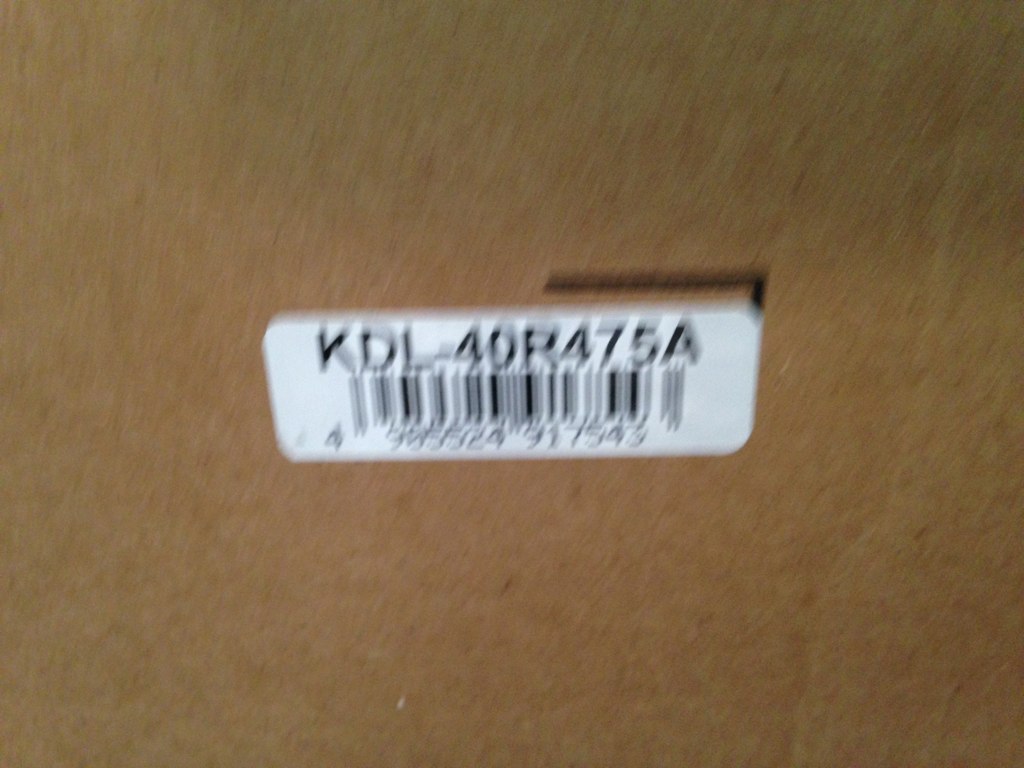A highly blurred close-up view featuring a barcode prominently displayed on a white label affixed to a cardboard box. Despite the blurriness, the barcode numbers are still legible. The label is strategically positioned at an angle on the box, indicating a design intended for precise scanning, likely by automated systems such as robots. The cardboard itself is a standard light brown, typical of regular packaging materials. Due to the extreme close-up nature of the image, the overall size of the box is indeterminable. The label contrasts with black lettering and barcode numbers, enhancing readability.